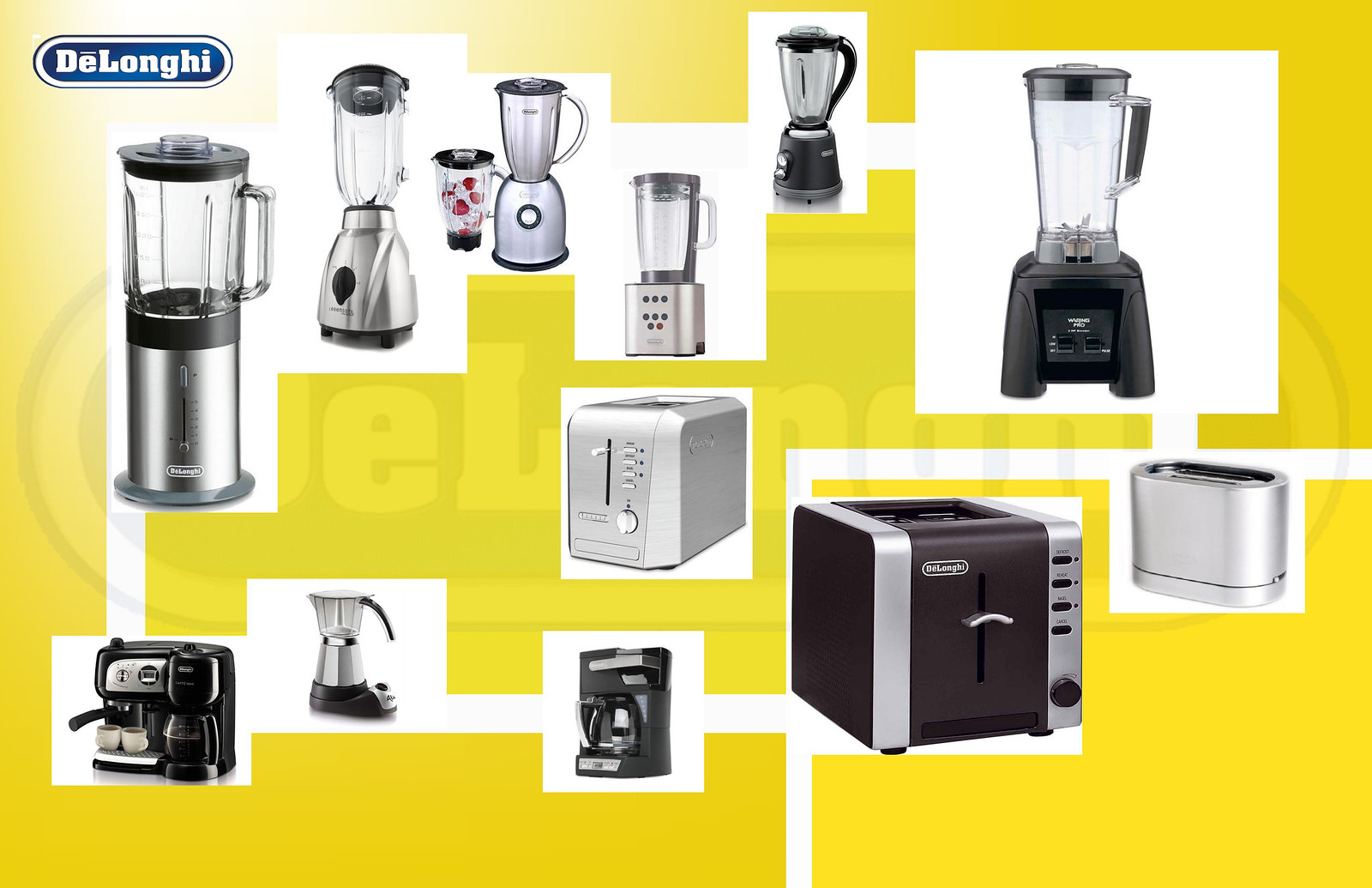The image showcases an array of DeLonghi kitchen appliances set against a yellow background with a white square embedded centrally. From the top left, under a blue oval with white "Delonghi" text, is a neat arrangement featuring six blenders. The blenders vary, with bases made of black plastic or silver metal, and clear blending tubes, some adorned with small, red strawberry designs. The blenders then transition to the mid-section, where the focus is on coffee makers positioned below the blenders. These include two black coffee makers, one resembling a cappuccino machine with two cups, and a silver coffee maker with traditional design. Finally, at the bottom section, there are three toasters displayed. Two are silver and feature sleek designs, while one is black, maintaining a more classic appearance. The black and silver theme of the appliances contrasts strikingly against the vibrant yellow backdrop, creating a visually appealing presentation of DeLonghi's kitchen products.